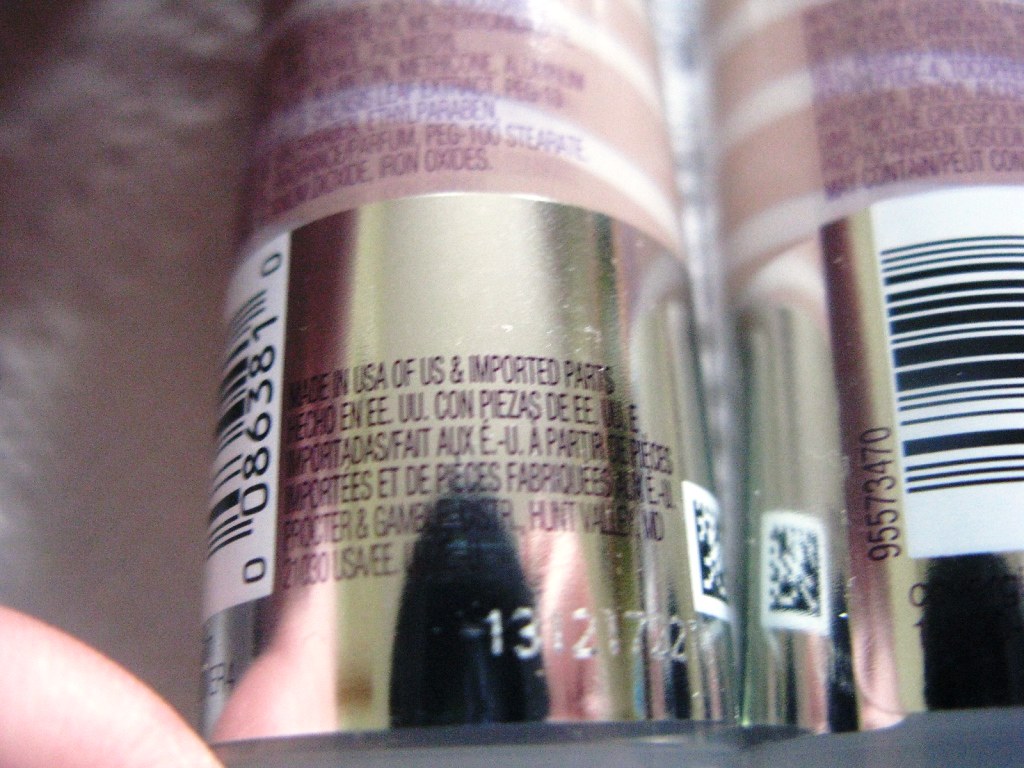The image features the back or bottom side of a packaging, though it's somewhat difficult to discern its contents due to the blurriness. The top part of the package displays a design of pink and white stripes, suggesting a potentially cosmetic or decorative product. The only legible text at the bottom reads, "Made in USA of US and imported parts," but its significance remains unclear. The package appears to be positioned near a mirror, as the same image is reflected on the opposite side. Alternatively, it could be two identical packages placed side by side.